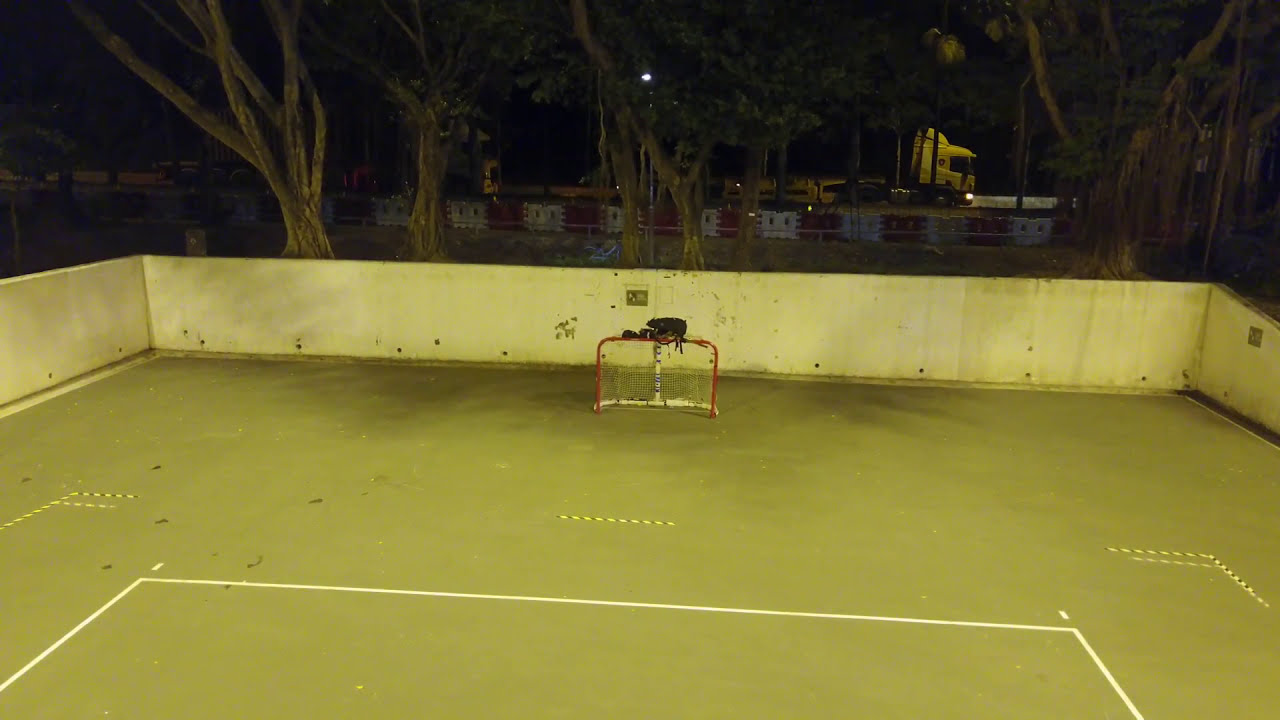This image captures a nighttime view of an ice rink without any ice, repurposed possibly for street hockey or rollerblading. Central to the scene is a red-framed goal with a white net, positioned directly in the center. In front of this goal, there’s a striking pattern on the light green ground: a series of yellow and black stripes arranged at various angles, forming a distinctive layout that includes a white rectangular line encompassing the area. Surrounding the rink is a barrier, predominantly white with yellow accents. Beyond this barrier, tall brown tree trunks and scattered vegetation stretch out into the background, accompanied by some buildings. The top of the image is enveloped in darkness, indicating the late hour. To the upper right corner of the frame, a yellow truck is visible, moving to the right. The rink itself and the adjacent area are illuminated by street lighting, casting a gentle glow across the entire scene.